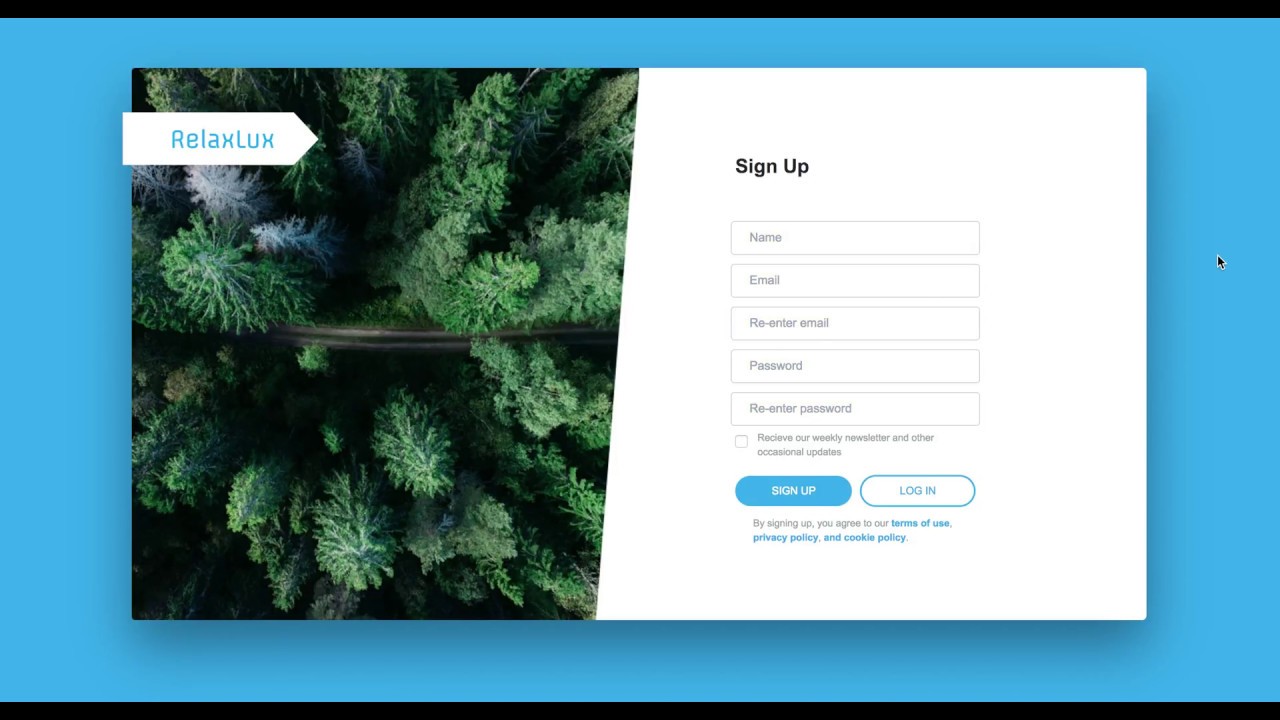The image features a multi-colored border, with thin black borders running horizontally across the top and bottom edges. The primary background color of the image is a light blue.

At the top left, there is a pop-up section labeled "Relax Lux," displayed in light blue text over a white pinned section. This overlay partially covers an aerial view of a forest, which prominently features a central pathway or road winding through the greenery.

To the right of this pop-up, there is a dedicated area with a white background, where a sign-up form is presented. The top middle of this section reads "Sign up" in black text. Below this title, there are several boxed fields arranged vertically for user input:

1. **Name**
2. **Email**
3. **Re-enter email**
4. **Password**
5. **Re-enter password**

Beneath these fields, there is an option stating: "Receive our weekly newsletter and other occasional updates," accompanied by a small checkbox for user selection.

At the very bottom of this section, two blue and white action buttons are displayed: 
- The left button is labeled "Sign up"
- The right button is labeled "Log in."

Overall, the image effectively combines a visually appealing background with a clear and user-friendly sign-up form.